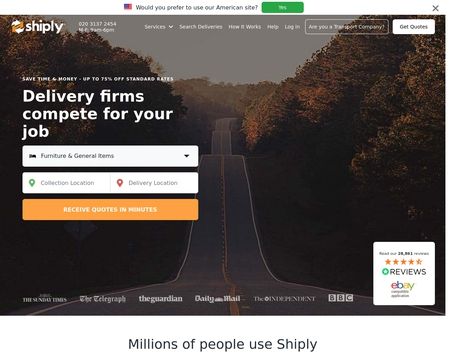Certainly! Here is a cleaned-up and detailed caption for the given image:

---

The image depicts the homepage of the logistics website, Shiply. At the top, a notification banner prompts users with the message: "Would you prefer to use our American site?" accompanied by a green "Yes" button. Below this, a scenic photograph of a winding, undulating blacktop road stretches into the distance, flanked by lush, green trees on either side.

In the corner of the photograph, the Shiply logo is displayed. Beneath the photo, a text overlay reads, "Save time and money up to 75% off standard rates. Delivery firms compete for your job." A drop-down menu titled "Furniture and General Items" allows users to specify their shipment type. Subsequent fields prompt for "Collection Location" and "Delivery Location," with an orange button labeled "Receive Quotes in Minutes" prominently placed in the center.

At the bottom of the photograph, several media logos are displayed, albeit with low resolution, including The Telegraph, The Guardian, Daily Mail, and BBC. In the bottom-right corner, a rating appears with "4.5 stars" next to an eBay logo, though the text is blurry and difficult to read clearly.